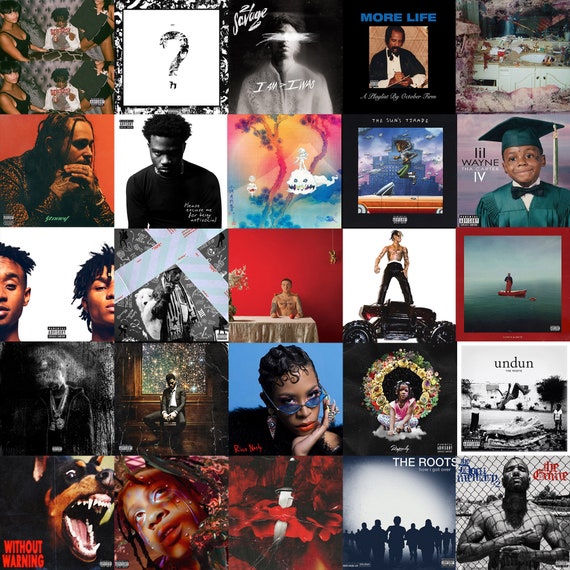The image depicts a grid of 25 album covers, primarily showcasing African American rap artists. Featured prominently are albums by The Roots, DMX, Lil Wayne, Jay Z, and 21 Savage. Each album cover varies in design, with many displaying the "Parental Advisory" warning in the bottom corner. The covers include diverse imagery: a person standing on tires, a kid in a graduation cap and gown, two men posing together, and a couple. The majority of these covers are from the 1990s onward, typically showing dark-skinned individuals. The collection is largely male-dominant, with only one album by a female black artist visible.